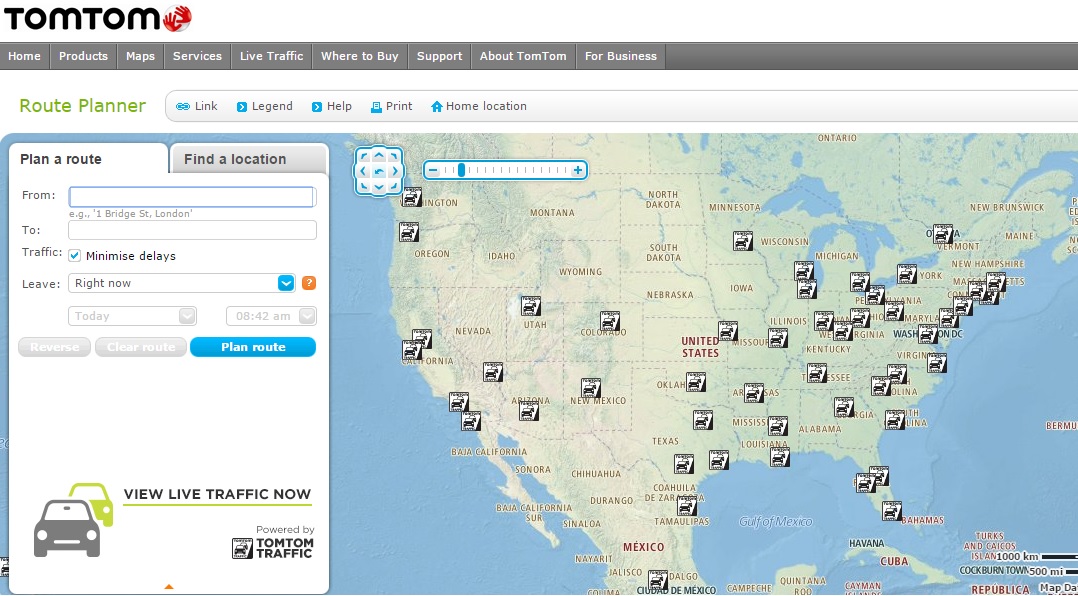This is a screenshot from the TomTom website, featuring the route planner interface. The user has specifically selected the route planner and customized it to display a legend, a help bar, a print option, and their home location. At this stage, the user has not entered their starting point or destination but has opted to minimize traffic delays and chosen the "leave now" option, indicating imminent travel plans. The interface and font style suggest that this is an older version of the TomTom website. The screen prominently displays a map of the United States on both sides, adorned with various icons depicting small cars within white and black squares, which likely represent possible travel destinations or TomTom-friendly locations.